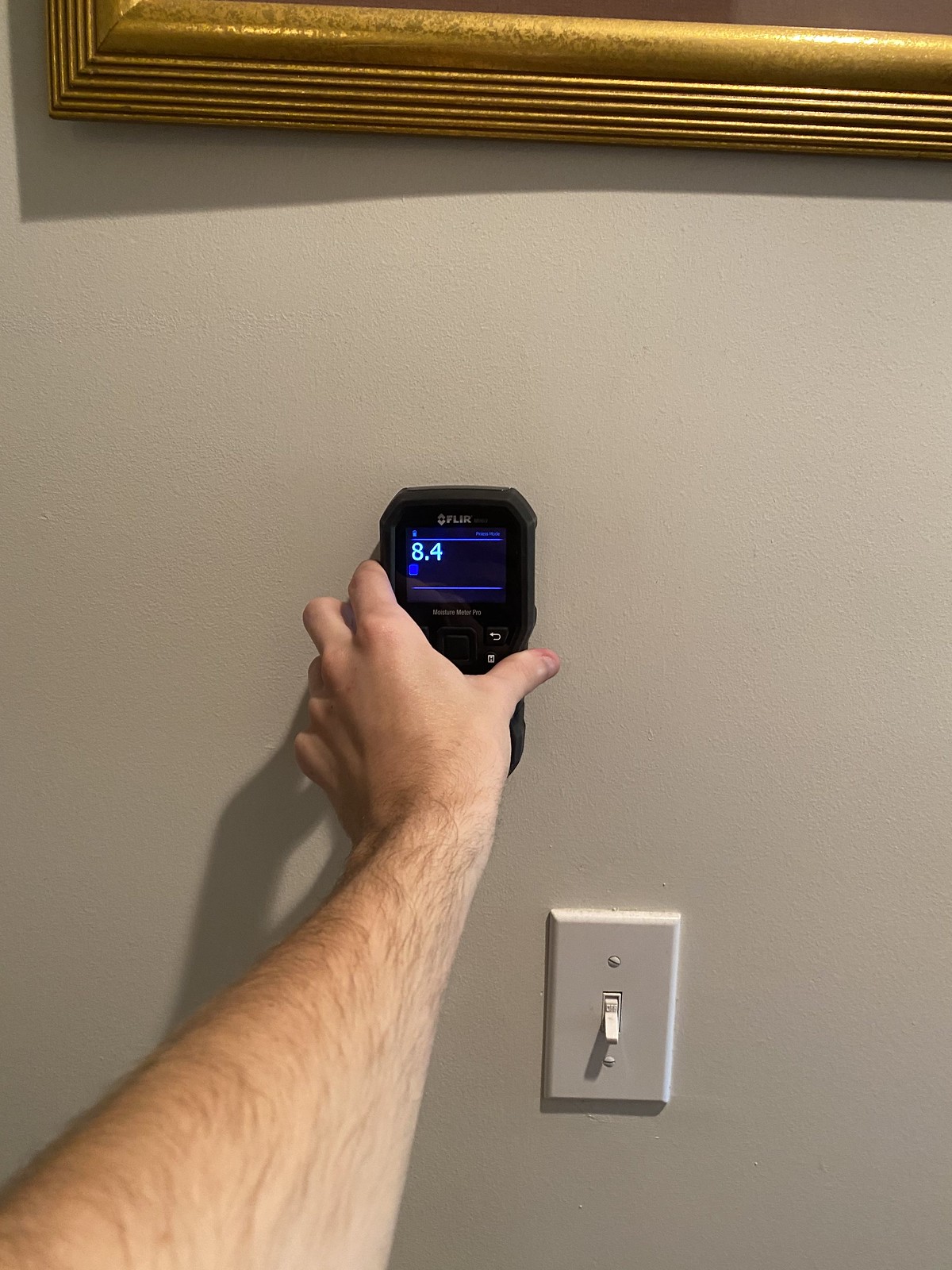In this detailed photograph, a white male with dark hair on his forearm is depicted holding a black stud or electrical current detector against a painted white wall. The wall, either weatherboard or gyprock, serves as the primary backdrop. Centered prominently in the image, the detector showcases a dark blue screen with navy blue lines and displays the number "8.4" in bright blue digits. The man's left arm, specifically his forearm, is visible as he maintains a firm grip on the device. Above the detector, the bottom edge of an ornate gold-framed picture frame peeks into view. To the bottom right of the detector, a standard white light switch, secured by two screws concealed with white plugs, is affixed to the wall, its switch pointing downward.